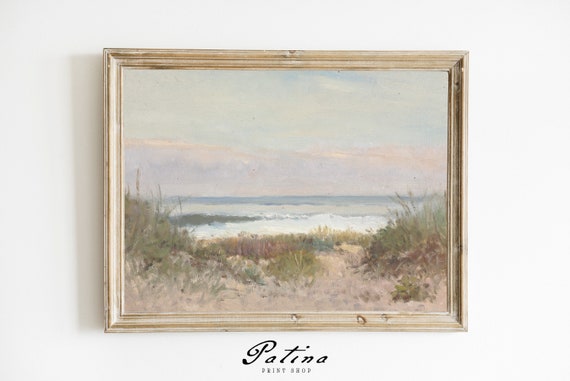Hanging on a pristine white wall, this artwork is evocatively presented in a light, possibly bleached wooden frame that subtly complements the freshness of the scene depicted within. The painting itself appears to be an exquisite oil painting, capturing a serene seashore landscape. A sandy dune, gracefully adorned with tufts of grass, dominates the foreground. Beyond the dune, a tranquil, sheltered bay extends into the background, shaped by a spit of land curving in from the left. Farther out, the bay gives way to the open ocean, where the horizon is lined with a delicate layer of clouds. The sky above is partially cloudy, revealing patches of blue that accentuate the calm, coastal atmosphere. Below the painting, "patina" is elegantly scripted, while "print shop" appears in clean, block type, grounding the artwork in an air of sophistication and craftsmanship.